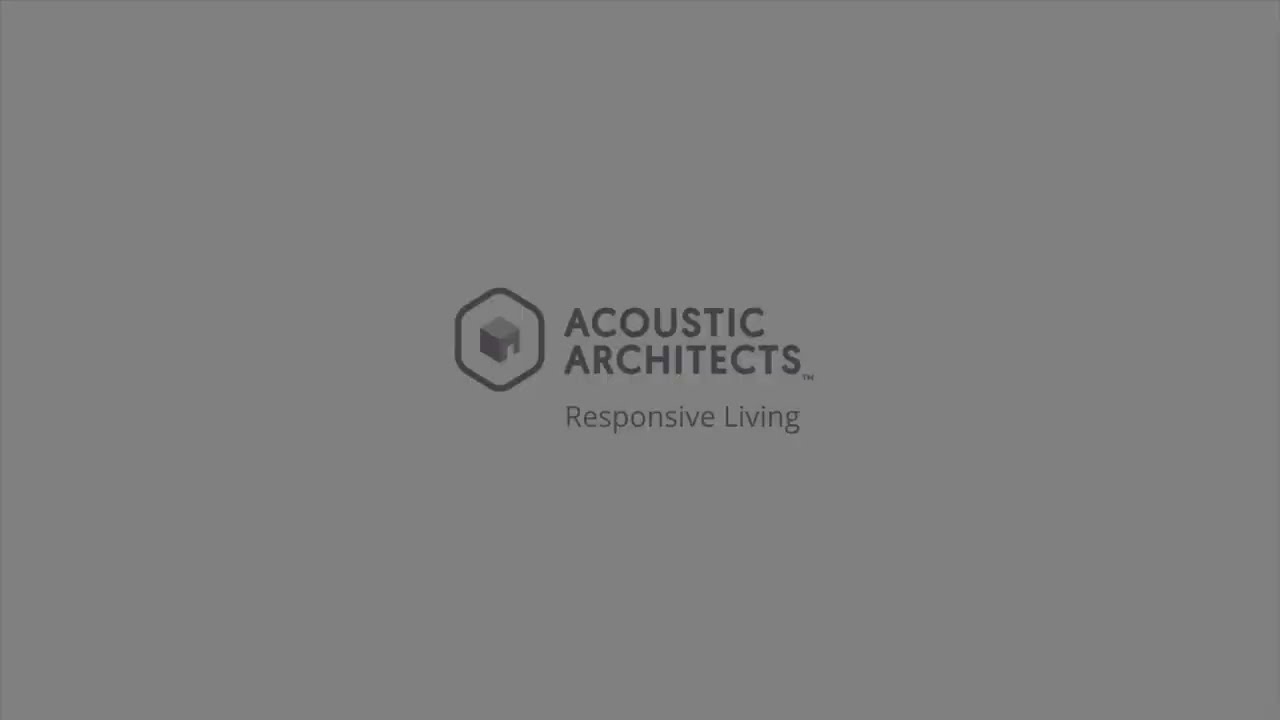The image is a minimalistic, professional graphic that appears to be an advertisement or promotional material for a company called Acoustic Architects. The background of the wide rectangular image is a solid light gray, almost twice as wide as it is tall. At the center of the image, in uppercase dark gray letters, the text "Acoustic Architects" is displayed, with "Acoustic" positioned directly above "Architects." A small trademark symbol is nestled under and to the right of the "S" in "Architects." Below this main text, in lighter gray and not bolded, is the company's slogan, "Responsive Living." To the immediate left of the central text is a logo: a dark gray, three-dimensional cube-like shape. This geometric figure contains a smaller, light gray cube inside it, with a tiny white portion that resembles an entrance, suggesting a structure or a house. The overall design is very simple, employing only different shades of gray, and it is devoid of any additional artwork or text, giving it a clean and professional appearance.